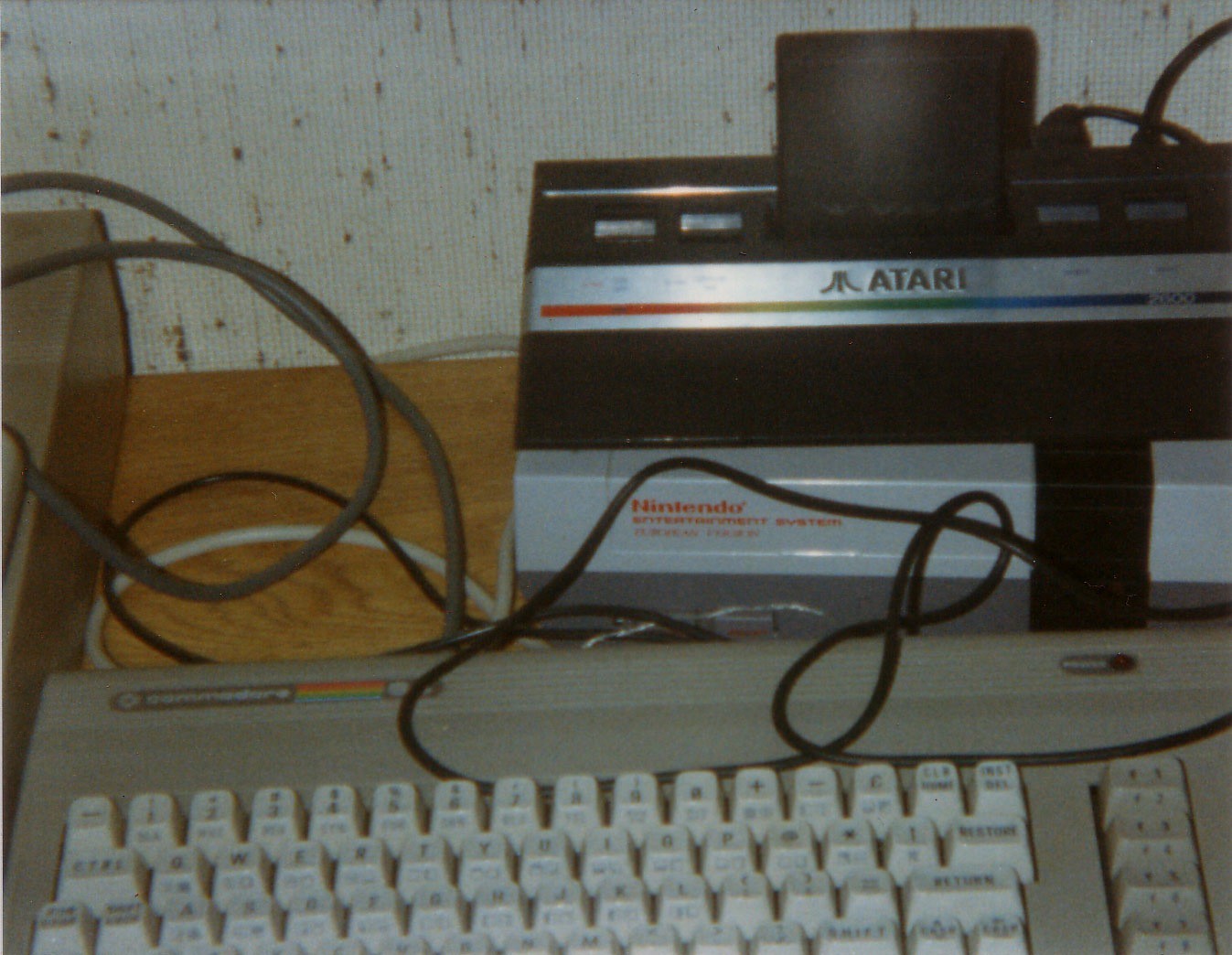The image showcases a vintage Atari play set prominently featuring the iconic "Atari" logo alongside text that mentions "Nintendo" and other illegible words. The backdrop is a white wall with irregular grayish blobs, adding a textured appearance. The Atari console is black with a distinctive silver bar on its front and additional silver detailing at the bottom. In the foreground, part of a gray QWERTY keyboard with white keys is visible, displaying its top three rows of keys. A noticeable tangle of cords extends from the game console to an unseen piece of equipment, adding a sense of nostalgic clutter. The overall scene is a blend of classic gaming elements and retro ambiance.